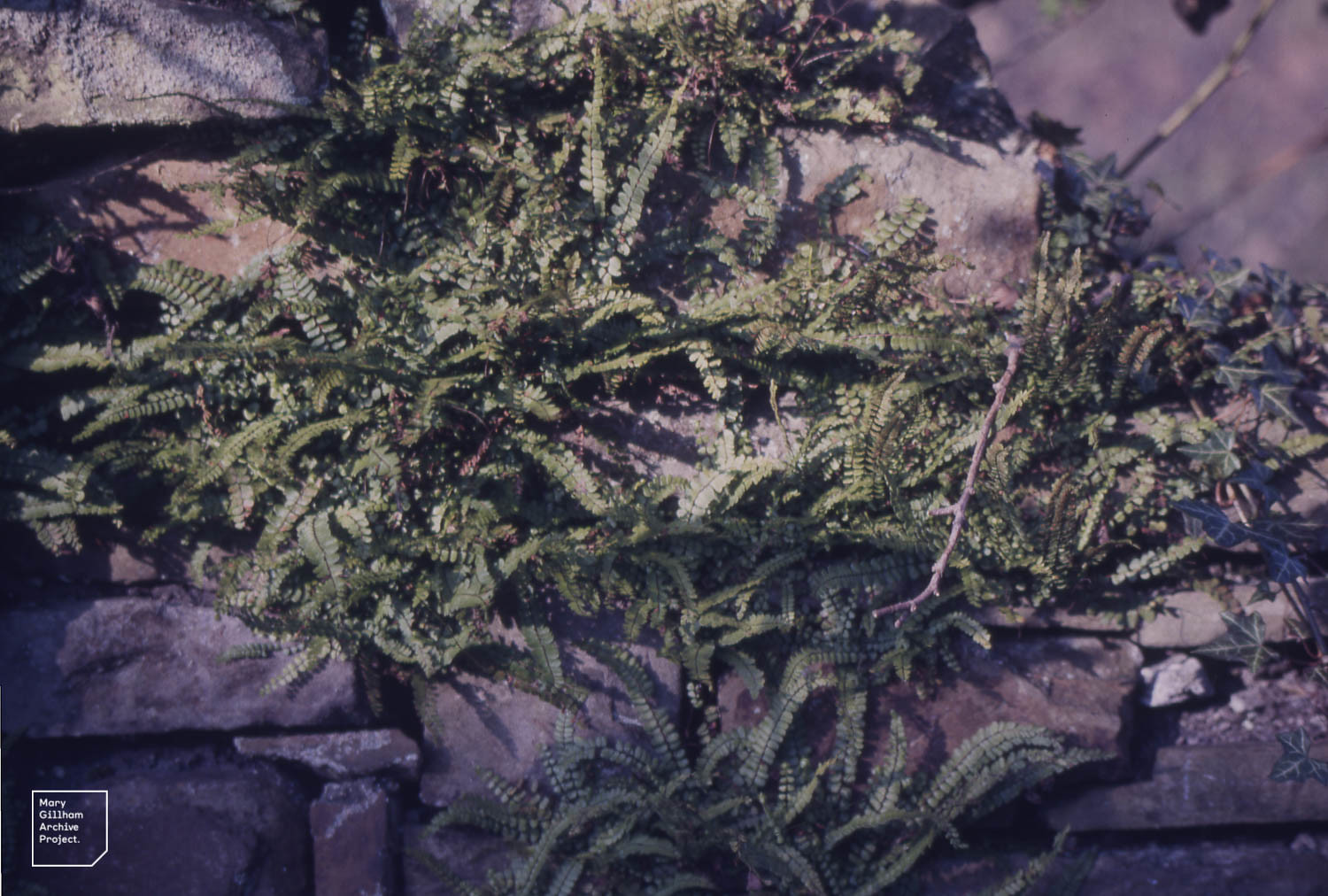The image displays a detailed photograph of a rocky surface covered with green, frondy plants and vines. The background showcases a gradient of light to darker purple hues, creating an almost otherworldly atmosphere. The scene includes clusters of large and small rocks, with approximately 70% of these rocks being overgrown by the greenery. Some rocks remain exposed, while twigs are scattered atop the vegetation. The gray, unusually smooth rocks and the peculiar posture of the plants evoke a sense of underwater ambiance, further accentuated by the visible shadows and eerie lighting. The positioning of the image is horizontal, and it features a logo on the bottom left corner stating "Mary Gilham Archive Project." Overall, the photograph beautifully captures the contrast of vibrant greens against the rocky and purplish backdrop, adding to its striking visual appeal.